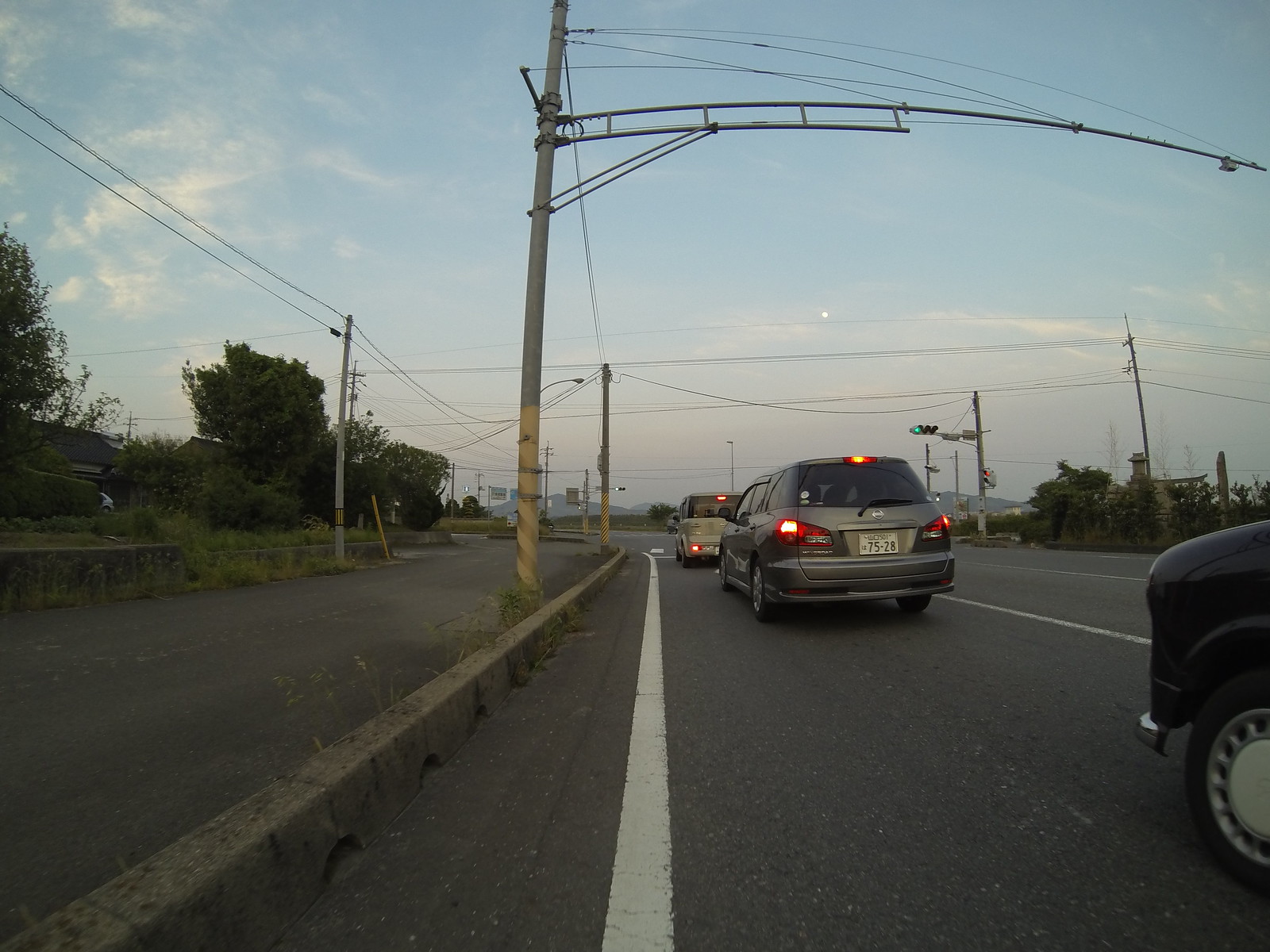The photograph depicts an urban intersection at dusk, with a light blue sky adorned with wispy white clouds and a visible moon. Centered on a solid white line marking the edge of the road, the image captures three cars: a silver minivan waiting at the traffic light, a black vehicle partially visible in the bottom right corner, and another car on the road. The traffic light shows a green indicator, suggesting cars are either stopped or starting to move. Electrical wires stretch above the road, connected by poles that line the kerb. Along both sides of the road, there are trees and green shrubs, with some weeds growing along the kerb. In the distance, the silhouette of industrial buildings is visible through a grey haze, adding depth to the urban landscape. Interspersed among these details are hints of a residential area, including what might be houses off to the left, and a pedestrian sidewalk.